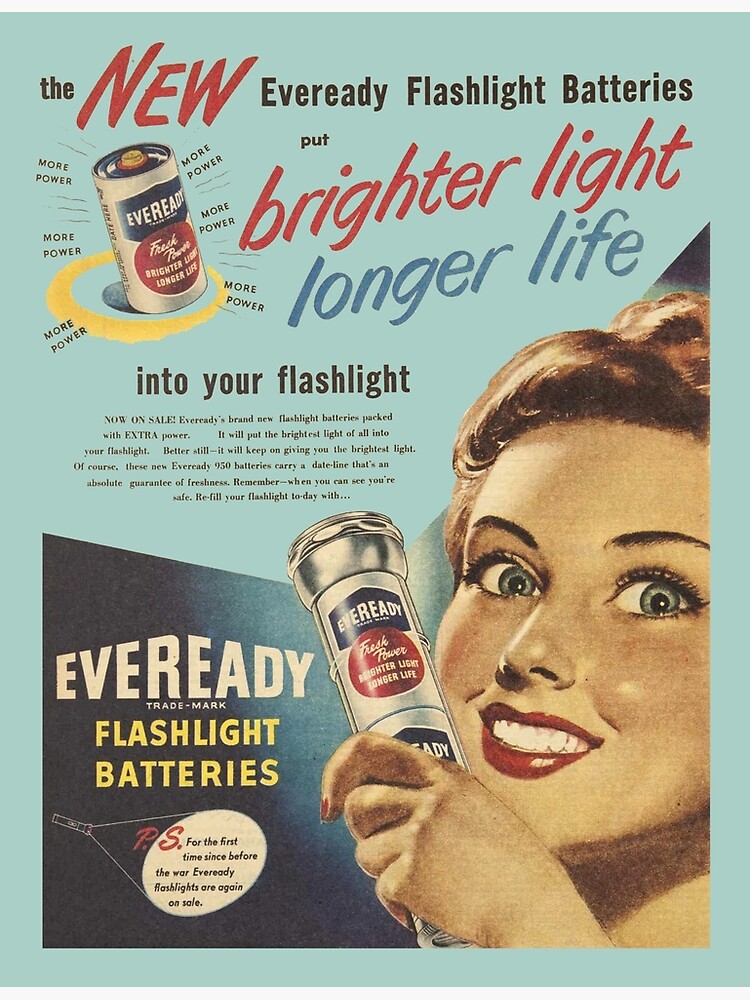The image is a vintage advertisement from the 1950s with a light blue background, promoting the new EverReady flashlight batteries. At the top, in large red letters, it reads "NEW," followed by "EverReady Flashlight Batteries." Below, it states in black text, "Put brighter light, longer life into your flashlight." Key phrases like "brighter light" appear in red text, and "longer life" in blue text. Central to the advert is a woman's face, featuring blue eyes, red lips, and a bouffant hairdo. She is holding a lit, silver EverReady flashlight in her left hand, which illuminates the text and an image of a cylindrical EverReady battery colored in white, blue, and red. Accompanying the visual is a yellow circle highlighting the words "More Power." The advertisement emphasizes that these batteries are back on sale with improved power and longevity for the first time since before the war, urging customers to refill their flashlights with EverReady for guaranteed freshness and reliability.